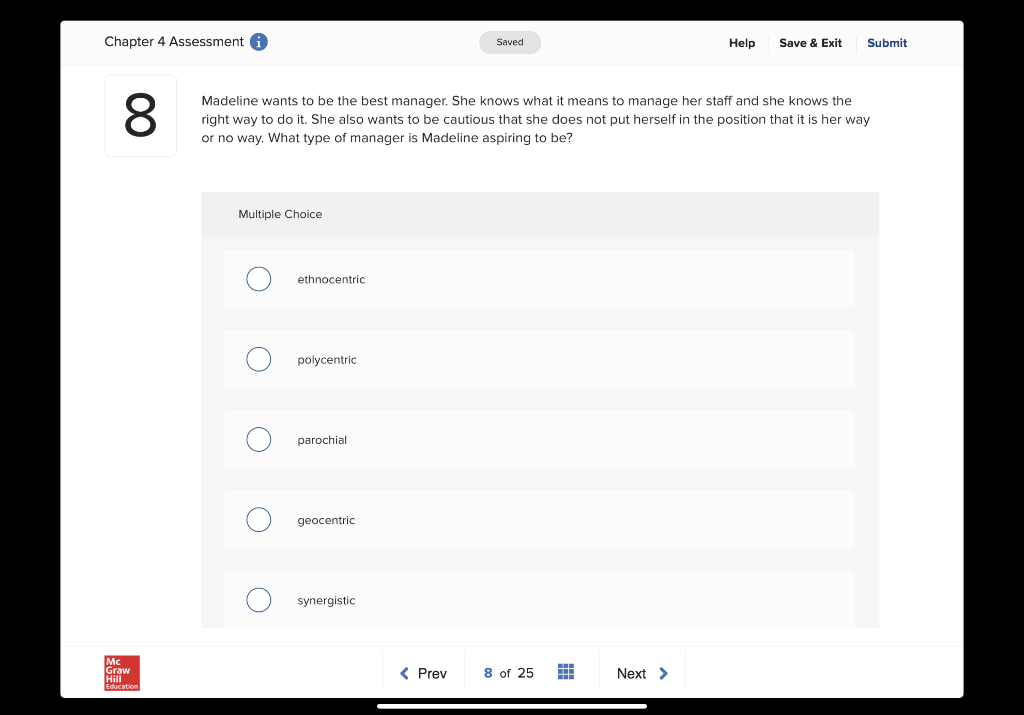Screenshot of a Chapter 4 assessment page from an educational software, likely a McGraw Hill platform. On the top right-hand corner, control buttons labeled "Help," "Save and Exit," and "Submit" are displayed. Dominating the center of the screen is question 8 out of 25, which reads: "Madeline wants to be the best manager. She knows how to manage her staff effectively and is aware of the importance of not imposing a 'my way or no way' approach. What type of manager is Madeline aspiring to be?" The question is followed by multiple-choice options: Ethnocentric, Polycentric, Paradoxical, Geocentric, and Synergetic. The software interface also shows navigation buttons at the bottom of the page: a "Previous" button with a left arrow, and a "Next" button with a right arrow. In the left-hand corner, a small red box with the McGraw Hill logo is visible, providing a clear indication of the assessment's source. Additionally, the navigation bar contains a square icon with nine small boxes, suggesting a menu or grid structure for switching between questions.